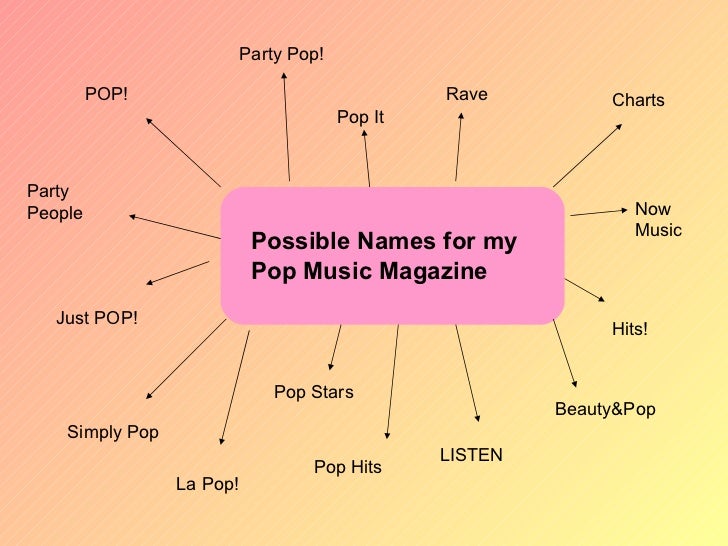The image depicts a vibrant idea board with a dynamic gradient background, transitioning from a yellow hue in the bottom right corner to a peach color in the top left corner, blending into shades of orange in the middle. Dominating the center of the image is a pink rectangle with rounded edges, containing the black text "Possible names for my pop music magazine." This central text is surrounded by various black arrows pointing outward in multiple directions, originating from the pink rectangle. These arrows vary in length and disperse to display potential magazine names in black text, including "Pop," "Party Pop," "Pop It," "Rave," "Charts," "Now Music," "Hits," "Beauty and Pop," "Listen," "Pop Hits," "Pop Stars," "La Pop," "Simply Pop," "Just Pop," and "Party People." The arrangement gives a sense of brainstorming, with the focal point and radiating ideas suggesting creativity and exploration in naming a pop music magazine.